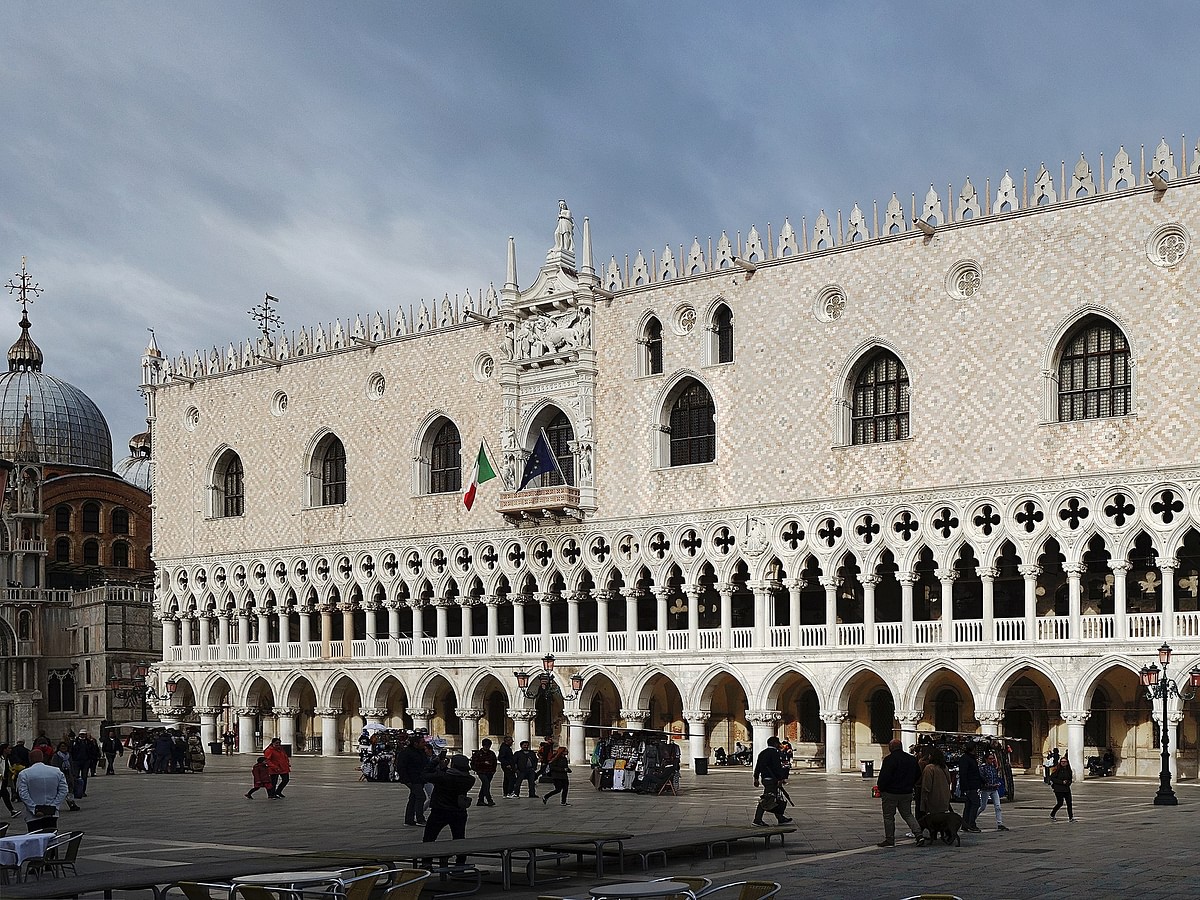This photograph captures the majestic facade of a prominent palace in Venice, Italy, set against a lively square bustling with people. The palace, marked by its large rectangular facade, features a visually striking diamond-shaped pattern with alternating stripes of tan and white on its upper portion. The lower section of the building showcases several light tan stone archways, with each arch topped by circles with cut-out cross-like symbols. Prominently in the center, there is an ornate balcony, perfect for addressing a crowd below, adorned with two fluttering flags: the vibrant green, white, and red stripes of the Italian flag, and a dark blue flag, possibly with gold stars, though its details remain unclear.

Above the balcony, a statue—likely a representation of a man or possibly a woman—stands with a dignified presence, surrounded by smaller decorative elements that resemble flames. The square in front is a hub of activity, populated with tourists and small vendor stands selling various goods, contributing to the lively atmosphere. To the left side of the palace, another impressive structure rises—a basilica crowned by a large dome with a cross atop, adding to the historic and cultural richness of the scene. The image conveys a sense of architectural grandeur combined with vibrant daily life, epitomizing the essence of Venice.